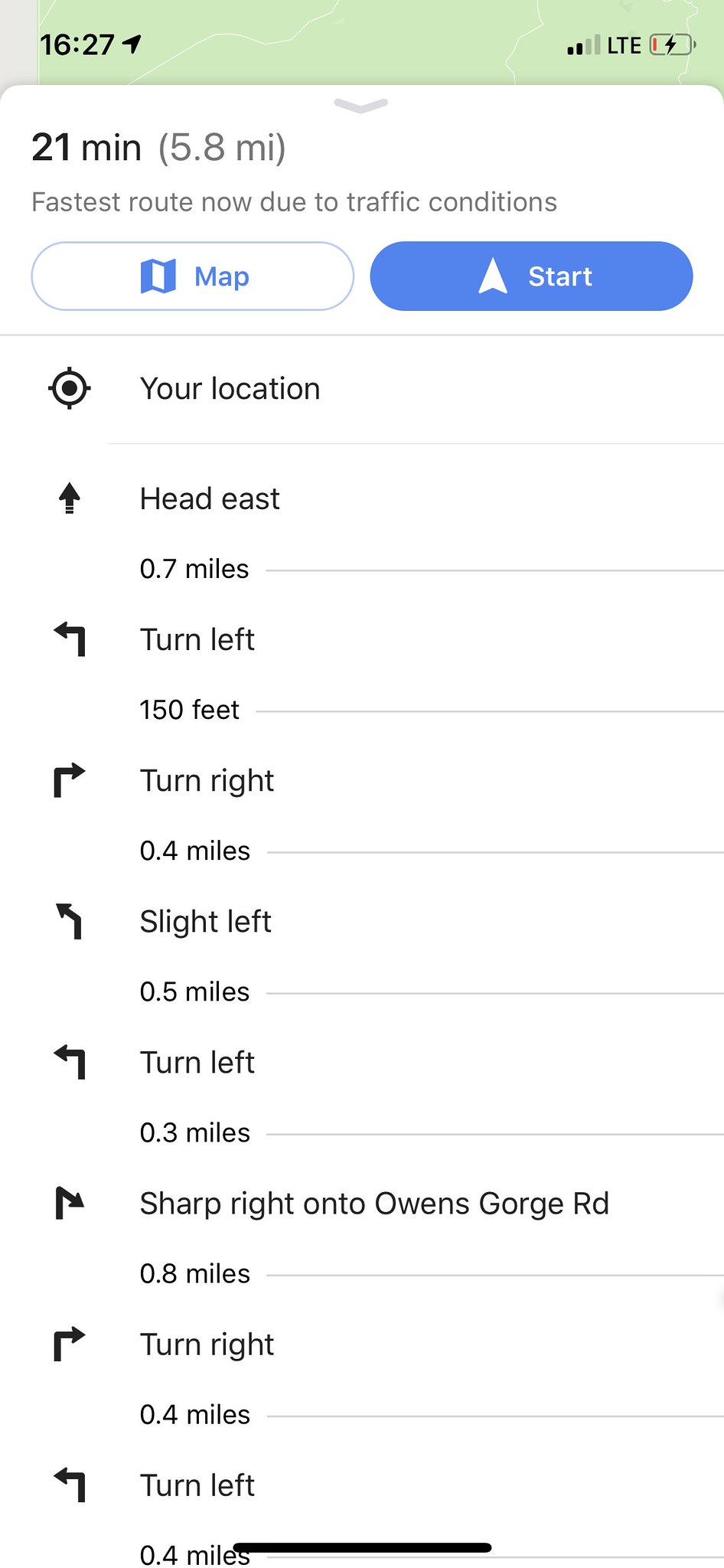The image depicts a Google Maps navigation screen on a mobile phone showing detailed directions from the user's current location. At the top, the time is displayed as 16:27, alongside an arrow indicating active navigation, with two bars of signal strength and an LTE connection. The battery icon shows critically low power. The route is 5.8 miles and estimated to take 21 minutes, marked as the fastest route due to current traffic conditions. There are two buttons: one to view the map and another blue button labeled "Start" for initiating navigation. The step-by-step directions include arrows for turning guidance: head east for 0.7 miles, turn left after 150 feet, turn right for 0.4 miles, slightly left for 0.5 miles, turn left for 0.3 miles, and take a sharp right onto Owens Gorge Road for 0.8 miles. Further instructions include a right turn after 0.4 miles and a left turn after another 0.4 miles. Each directional command is accompanied by corresponding arrows, and a scrollable bar at the bottom suggests navigation continuity for subsequent steps.